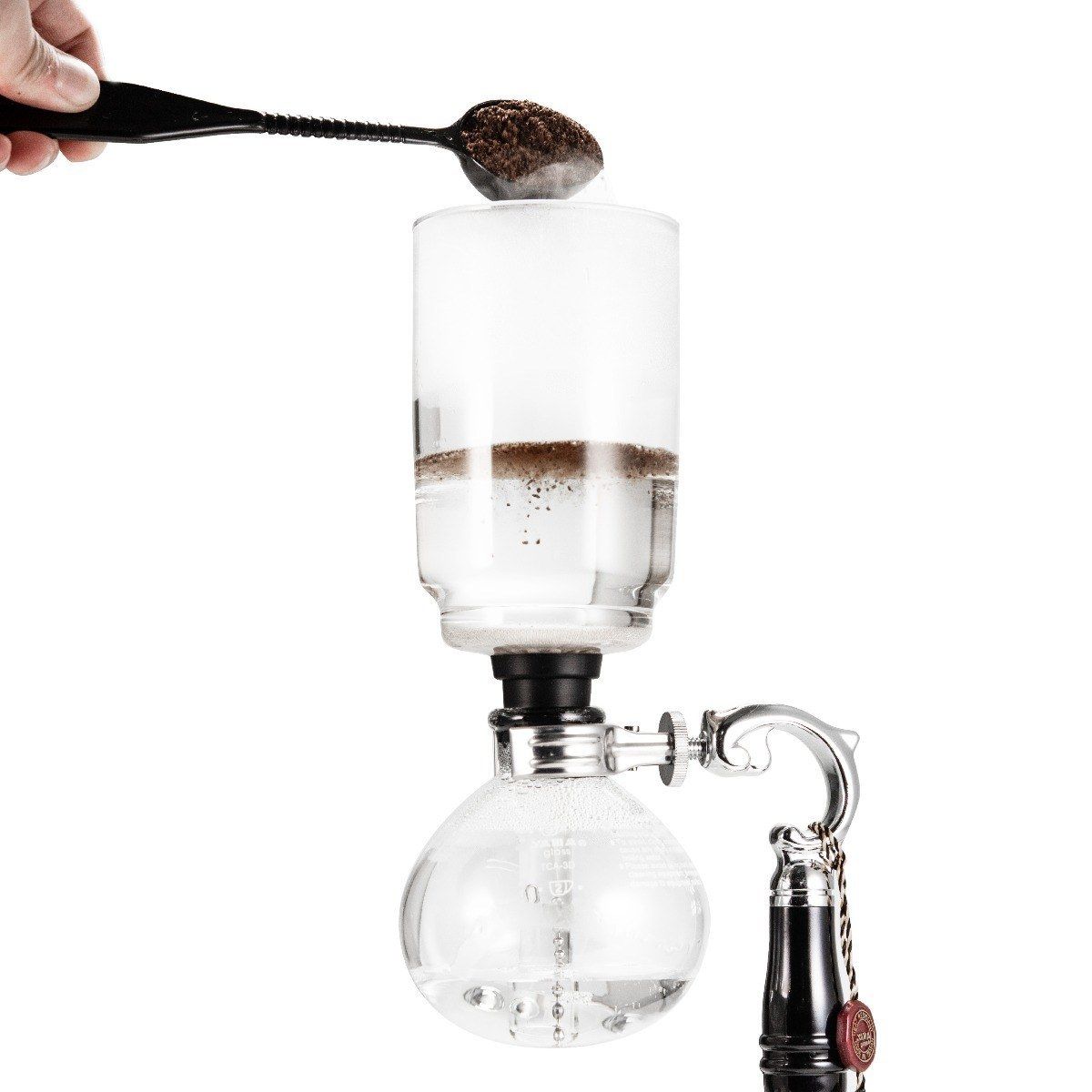This image features a horizontally oriented photograph with a stark white background. Dominating the center is an intricate glass apparatus, resembling a coffee or tea brewing device. The lower part of the setup comprises a glass bulb, distinguished by a slightly burnt or darkened bottom area, possibly indicating prior use. This bulb connects to an upper glass cylinder through a sleek steel sleeve. The top section is partially filled with a liquid, likely hot water, as suggested by its appearance and the steam rising from it.

On the left-hand side of the image, an outstretched hand holds a black spoon over the upper glass cylinder, depositing a substance, probably coffee grounds or tea leaves, into the hot water. The contents are visibly falling from the spoon, emphasizing the brewing process. Adjacent to the steel sleeve, there’s a distinct feature—a black handle with a metal loop or fitting, designed for easy handling or perhaps to regulate the device’s mechanism.

Overall, the glass apparatus portrays an ornamental and functional brewing device, likely used for making coffee or tea, rather than a piece of scientific equipment. The detailed elements, such as the black handle, the descending grounds, and the double-layered glass construction, highlight the elegance and utility of this beverage-steeping tool.